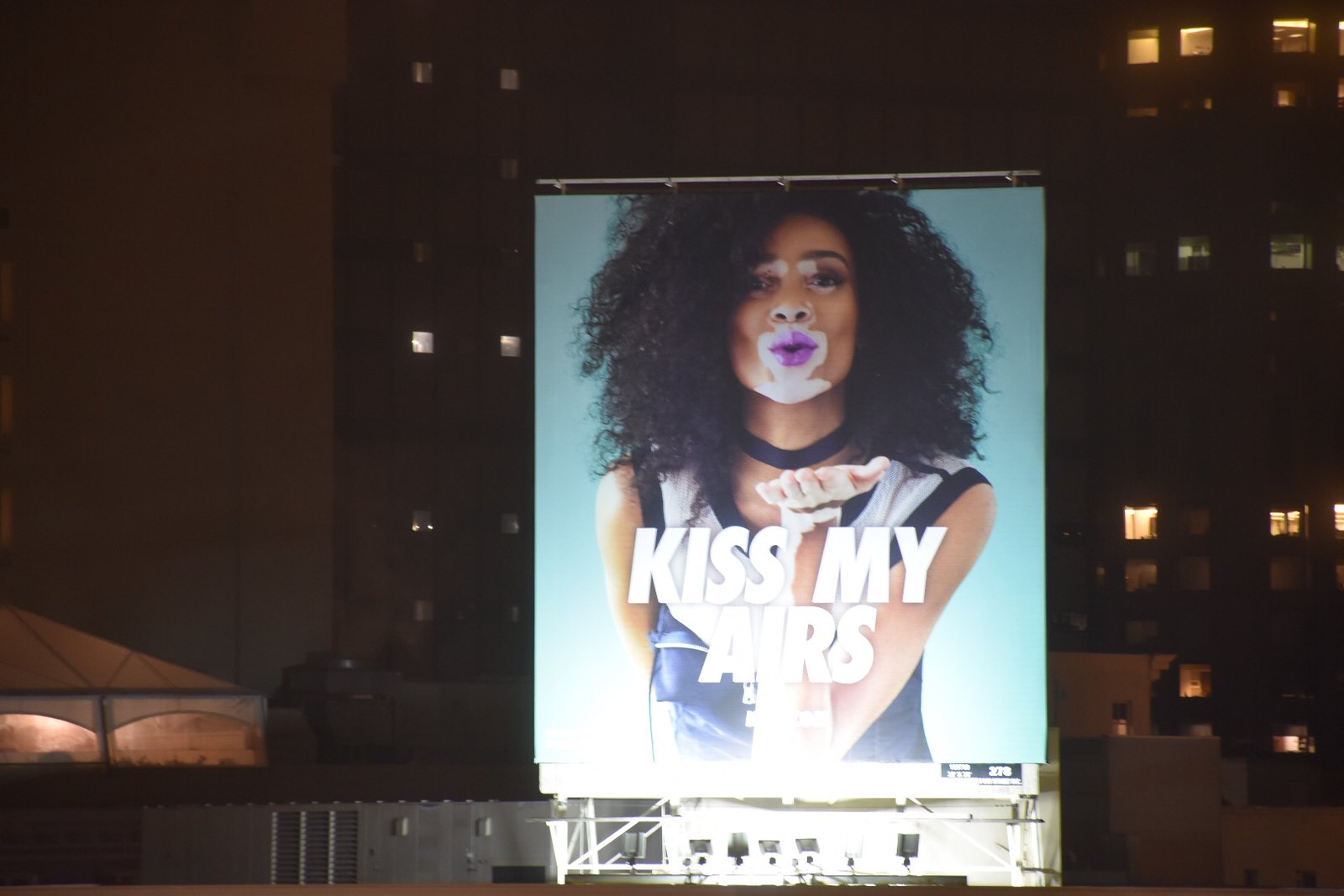In this nighttime photograph, a billboard takes center stage against a backdrop of city buildings with scattered illuminated windows. The billboard is lit from beneath by a series of spotlights, creating a striking visual against the deep blue sky. It displays an advertising image featuring a woman with an afro hairstyle and dark black curly hair. She has light brown skin with distinct white vitiligo markings around her lips, nose, eyes, hands, and shoulders. Wearing a sleeveless shirt with thick black trim, a black choker necklace, and purple lipstick accentuated with white outlining, she gestures as if blowing a kiss. The large white text on the billboard reads "Kiss My Airs." Below the billboard, a low white brick building with dark edging is partially visible, and to the left of the image, a white tent illuminated from within adds to the urban night scene. In the background, tall dark buildings rise, contributing to the cityscape, while lines or cables are seen stretching across the left side of the picture.